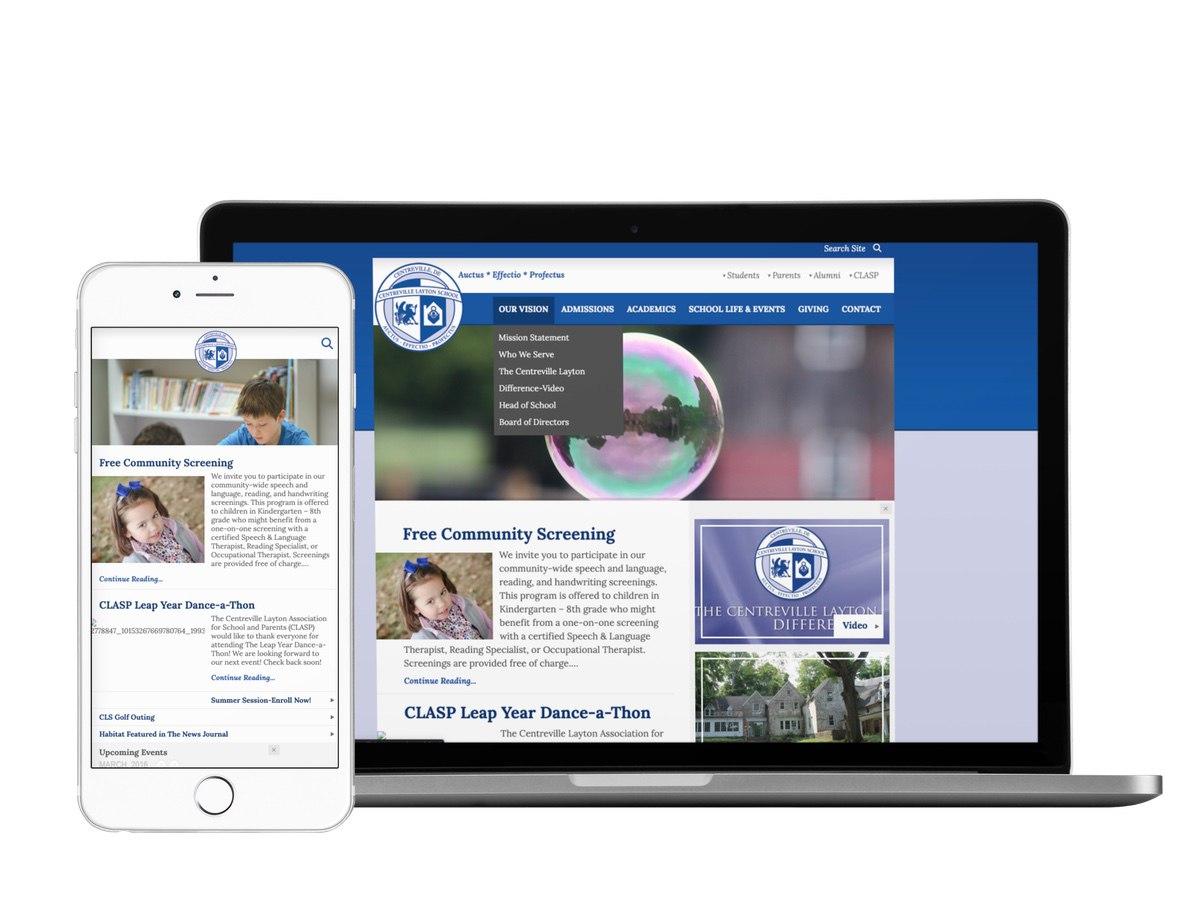The image showcases two electronic devices side by side: an older model iPhone and a laptop computer of unidentified make and model. Both devices are displaying the same community-focused website, which features a primarily blue background. The content visible on the screens is related to various community activities or events, with article titles such as "Free Community Screening," "CLASP," "Leap Year," and "Dance-a-thon." Additionally, the website includes images of young children. Despite the small text, the website appears to be affiliated with a foundation or community organization dedicated to outreach and events.